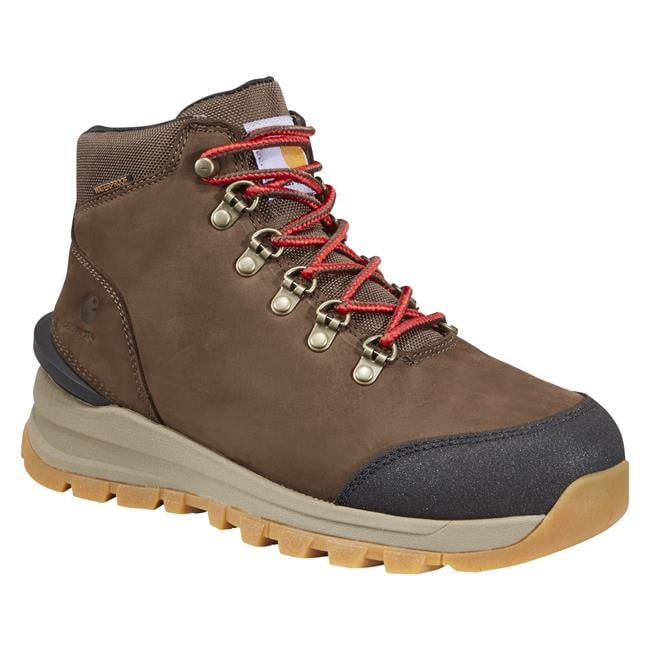The image is a color landscape photograph depicting a brown leather Carhartt hiking/work boot, prominently displayed with a backdrop that has been dropped out, giving the illusion that the boot floats against a white background. The boot, an ankle-high style, points its toe towards the bottom right corner and its heel towards the left. Distinguished by its meticulous details, the boot showcases a black toe box and heel accents, with metallic eyelets for the orange and brown laces. A white label featuring the Carhartt logo in gold is visible beneath the laces on the tongue, and a small side tab on the left proudly states "waterproof." The cream-colored sole is wedge-shaped, higher at the heel than at the toe, and features a robust, waffle-edged tread in light brown, wrapping around the front. The boot’s padded collar ensures comfort, while the Carhartt logo is embossed on the leather heel, reaffirming its brand and quality. The overall photographic style is highly realistic, emphasizing product photography and representationalism, capturing every nuanced feature of the boot.